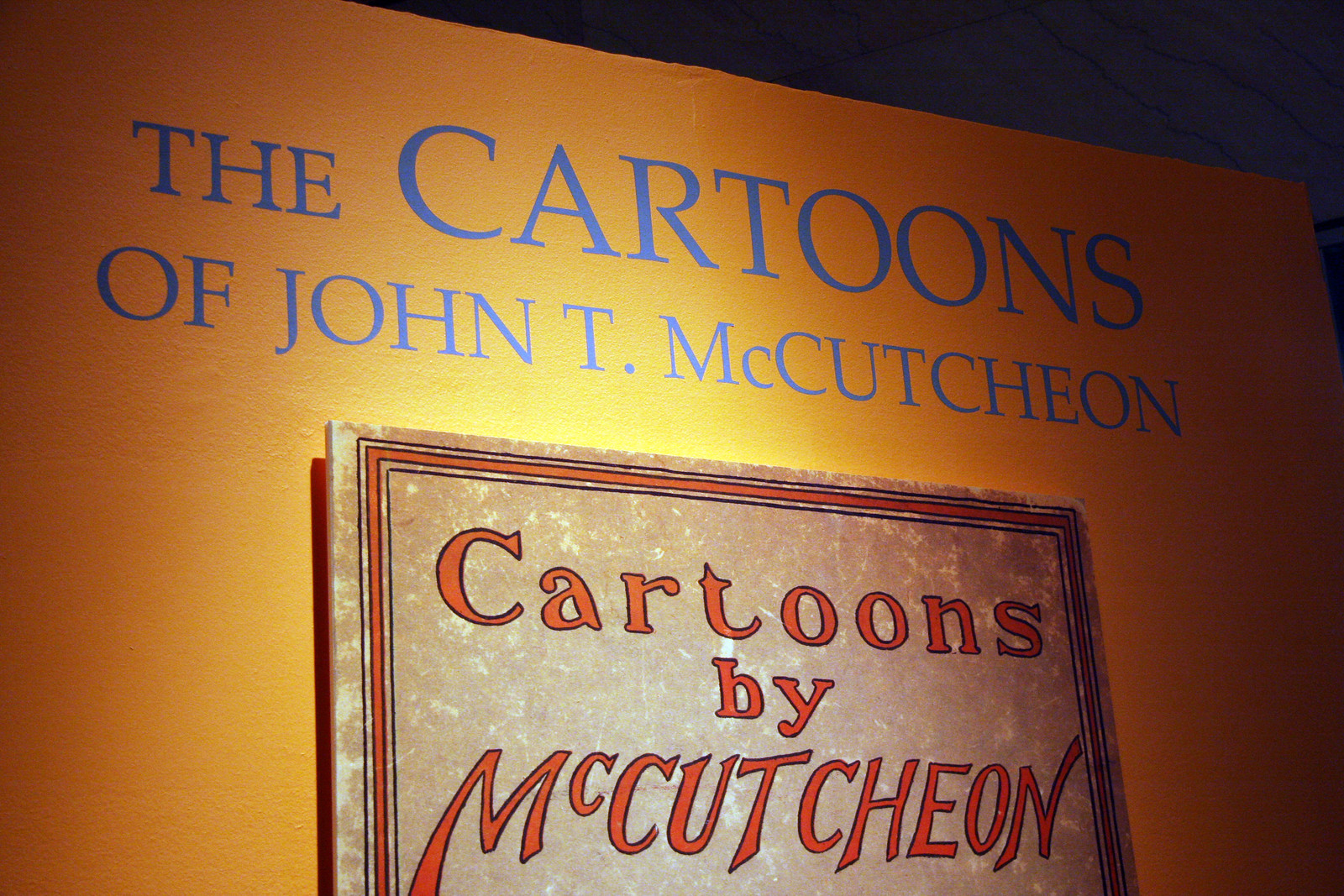Displayed prominently in a museum exhibit, a large sign titled "The Cartoons of John T. McCutcheon" catches the eye with its bold blue letters against a dark yellow background. The exhibit is set in a dimly lit room, with focused lighting illuminating the sign from above. Below the main title, an aged, brownish-white paper with worn edges features the phrase "Cartoons by McCutcheon" in striking red letters, framed by black and red trim. The sign and paper, exuding a vintage and cartoonish aesthetic, are mounted on an orange wall, which adds a vibrant contrast to the display. The overall setup, reminiscent of historical or artistic displays, hints at the significance and nostalgia associated with McCutcheon's works.